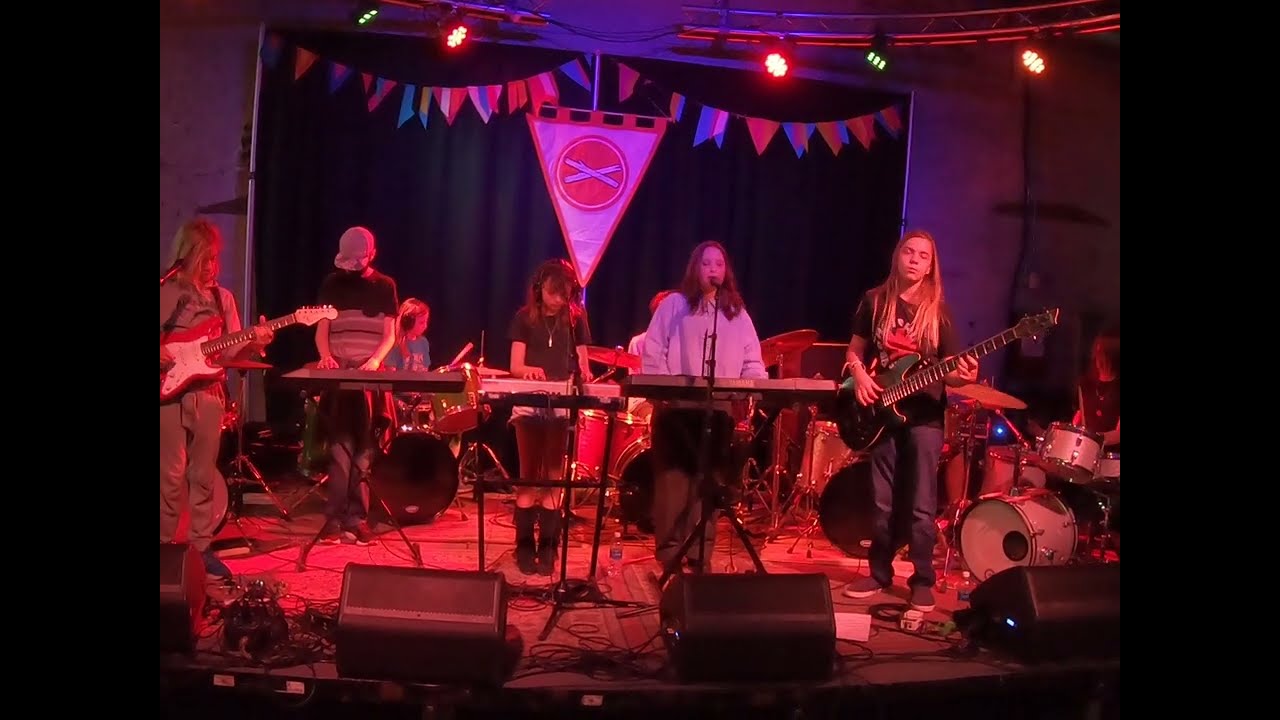A vibrant, detailed image captures a lively band performing on a crowded, rudimentary stage illuminated with red and green lights. The colored lights create a striking red glow that highlights the band members and their instruments. From left to right, the band consists of five visible members: a guitarist in jeans and a gray shirt, three keyboardists in the center, and another guitarist with long blonde hair on the far right. The central right keyboardist, who is also singing into a microphone, sports a white sweater. The middle keyboardist with a black shirt appears to be wearing headphones, and another keyboardist with their head down is wearing a hat. A mostly obscured drummer is positioned in the far right shadows. The stage features four speakers at the front and a backdrop adorned with colorful banners, possibly depicting crossed sticks. The presence of two black vertical bars running down both sides of the image frames the dynamic scene.